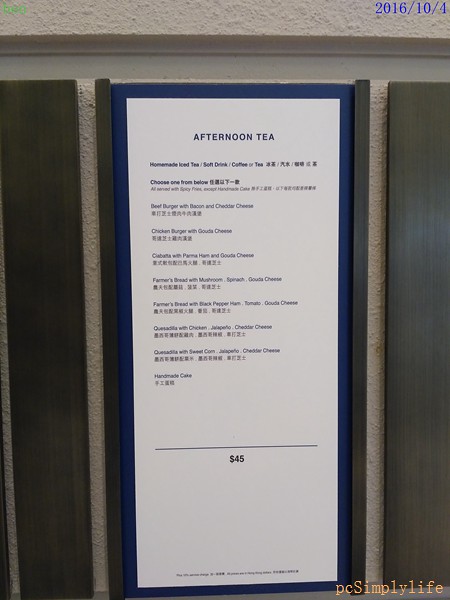The image showcases a meticulously framed menu displayed on what appears to be an interior wall. The menu itself is long and white, framed with a striking blue border. It resembles the length of two standard sheets of paper stacked vertically. 

In the backdrop, the wall is characterized by a white stripe across the top of the photo, leading into a thick tan segment that appears to be made of concrete or stucco. A blue date stamp at the top reads "2016/10/4," indicating either October 4th or April 10th, depending on the country.

The menu is being held up by what seems to be painted steel or wood. On either side of the menu, there are thin strips, and further out on both the left and right, there are broader strips of the same material. 

At the bottom of the image, a digital stamp reads "PC Simply Life," and the menu is specifically for afternoon tea. Although the text on the menu is mostly too small to discern, it appears to list a prefix menu with several lines of offerings. Two-thirds down the menu, a notable line highlights a price of $45, with very tiny writing also present along the bottom.